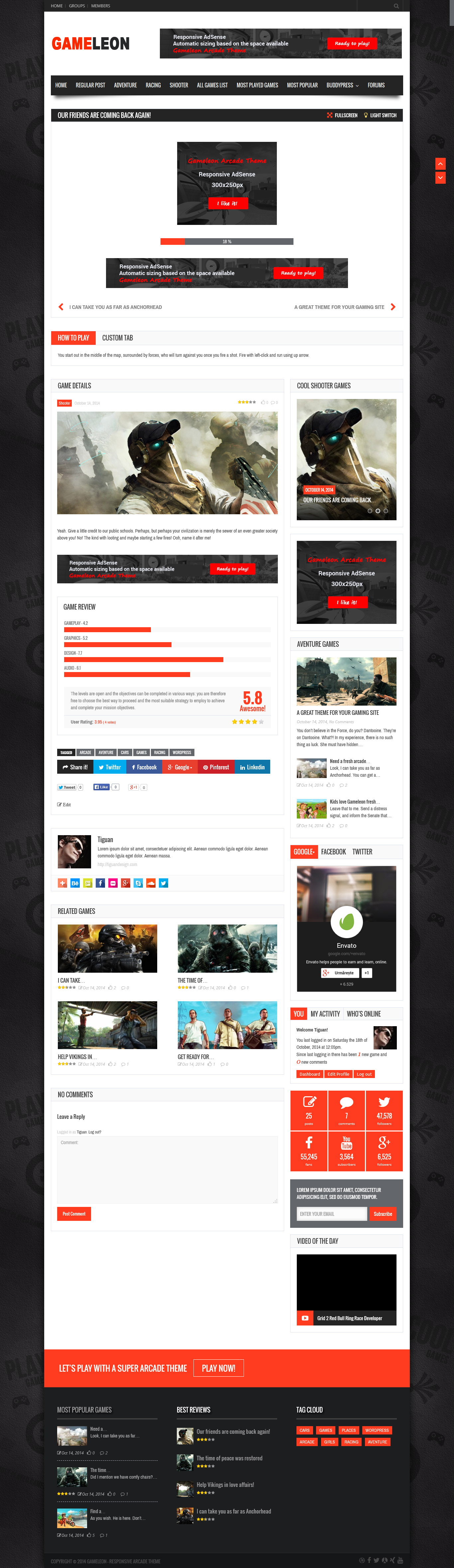Screenshot of a mobile device screen displaying the Game Leon website. The interface features a predominantly black background with a palette of red, black, and white elements. In the upper left-hand corner, the site’s logo reads "Game" in red and "Leon" in black, indicating a gaming-related website.

The primary content area includes a prominent vertical white bar listing various website information amidst a red, black, and white theme. At the top, there is an unreadable menu bar followed by a black, white, and red advertisement. Below this, another ad includes a prominent red button, suggesting a fundraising initiative.

Central to the page is a game review section for an unspecified post-apocalyptic game, rated at 5.8 on average. The game appears visually rich with an image of a soldier in a dystopian cityscape, notable for his bionic blue eye, baseball cap, earpiece, bandana-covered face, camouflage uniform, and distressed American flag. Adjacent to this are functionality buttons such as "How to Play" and "Custom Tab."

Along the right sidebar, there's a "Cool Summer Games" list with adventure game tiles and social media icons for Facebook and Twitter. The sidebar also shows user profile and activity details, a list of online users, a social media tile, a search or subscription box, and additional navigation elements.

The bottom of the screen features further content including "Most Popular Games" with three game listings, "Recent Reviews" showcasing four reviews, and a tags section for site navigation. No comments are present at the bottom, with an option to leave a reply.